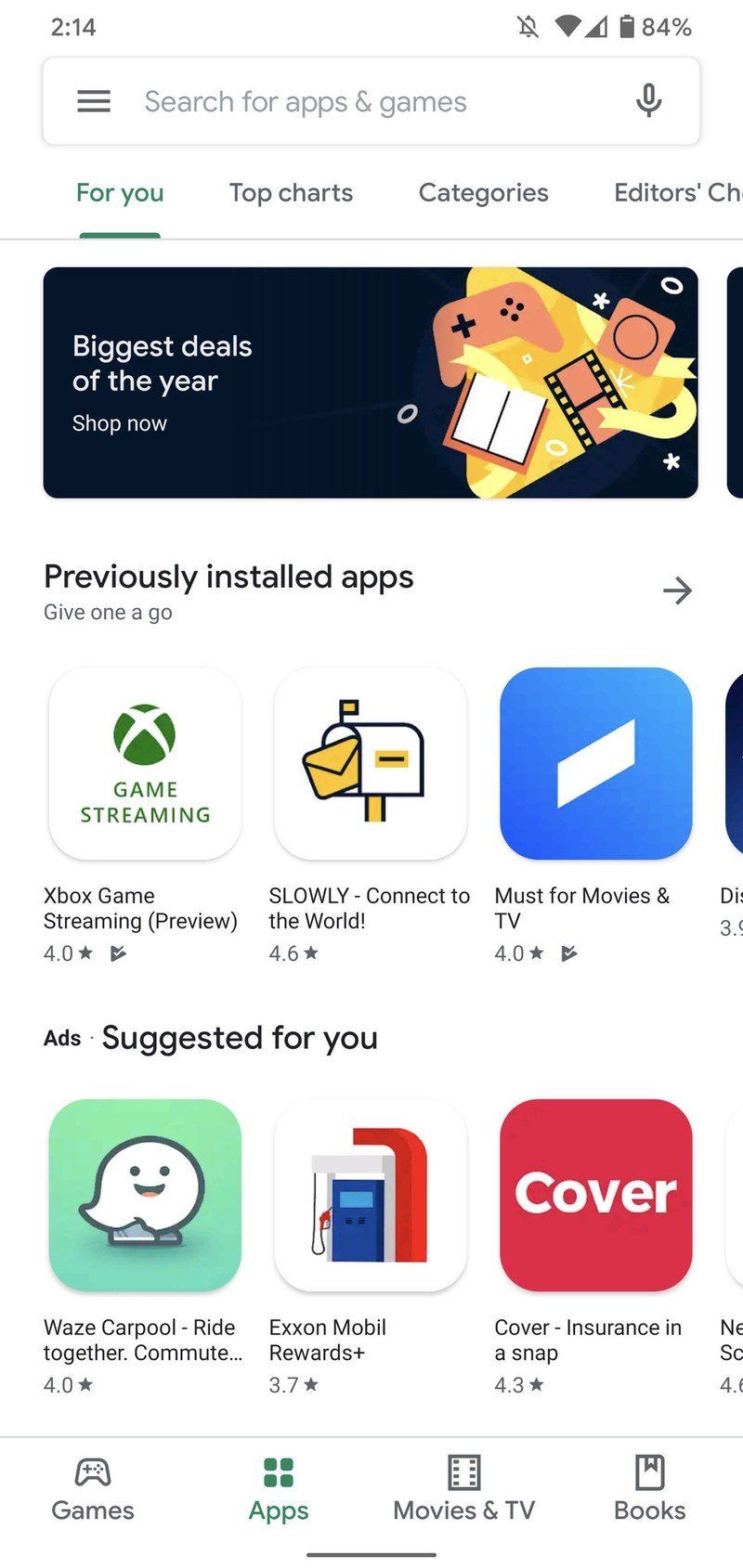In the Google Play Store on a smartphone, the screen displays a search bar at the top, ready for queries. Below the search bar are main sections like "For You," "Top Charts," "Categories," and "Editor's Choice." A promotional banner labeled "Biggest Deals of the Year" encourages users to shop for premium deals. The interface features a sleek black background adorned with icons, including a game controller and film stock, adding a touch of modern and vintage charm.

Scrolling further, the screen showcases a list of previously installed apps. Among these are "Xbox Game Streaming," a must-have for gaming enthusiasts, and "Slowly," a social app that connects users across the world. Another notable app is "Connect," which is essential for TV and movie aficionados.

Advertisements personalized for the user are clearly labeled "Suggested for You." Featured apps include "Waze," which displays a cheerful ghost icon, and "Exxon Mobil Rewards," symbolized by a gas pump. The app "Cover" promises insurance in a snap with its intuitive interface.

The background of the screen is white, creating a clean and organized layout. At the bottom navigation bar, users can access sections such as "Games," "Apps," "Movies & TV," and "Books." The current focus is on the "Apps" section. Each app is represented with a distinct icon; for example, "Waze" features a smiling ghost, "Exxon Mobil Rewards" has a gas pump icon, and the Xbox app proudly displays the Xbox logo.